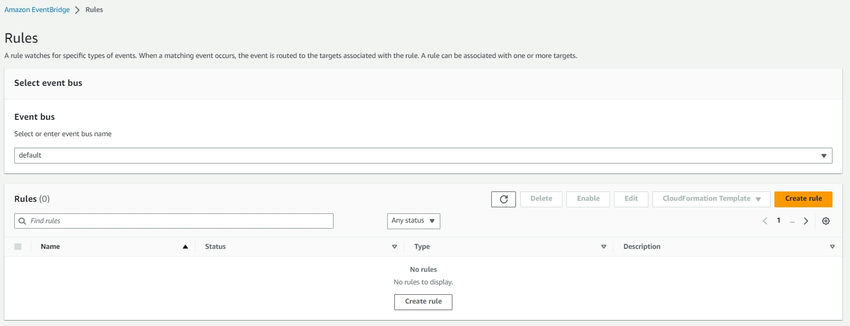A screenshot captures the interface of the Amazon EventBridge scheduling app, a serverless solution designed to create, run, and manage tasks from a centralized location. The background features a gray hue. 

At the top-left corner, "Rules" is prominently displayed in large, black letters, with a brief description below in smaller, black text. Directly underneath, a large gray box contains the text "Select event bus" in small black letters, accompanied by a drop-down box currently set to "default."

On the bottom-left, "Rules" is again written in bold, smaller black letters, with a parenthetical note indicating "(0)." Below this, a search box labeled with "Find sales" is present. The columns labeled "Name," "Status," "Type," and "Description" remain empty.

In the center of the interface, a message reads "No rules," above which a prominent white box with the text "Create rule" is situated. Toward the right-center area, several buttons are aligned: "Refresh," "Delete," "Enable," "Edit," and a drop-down box. An orange button labeled "Create rule" stands out. Most elements are grayed out except the "Refresh" and "Create rule" buttons.